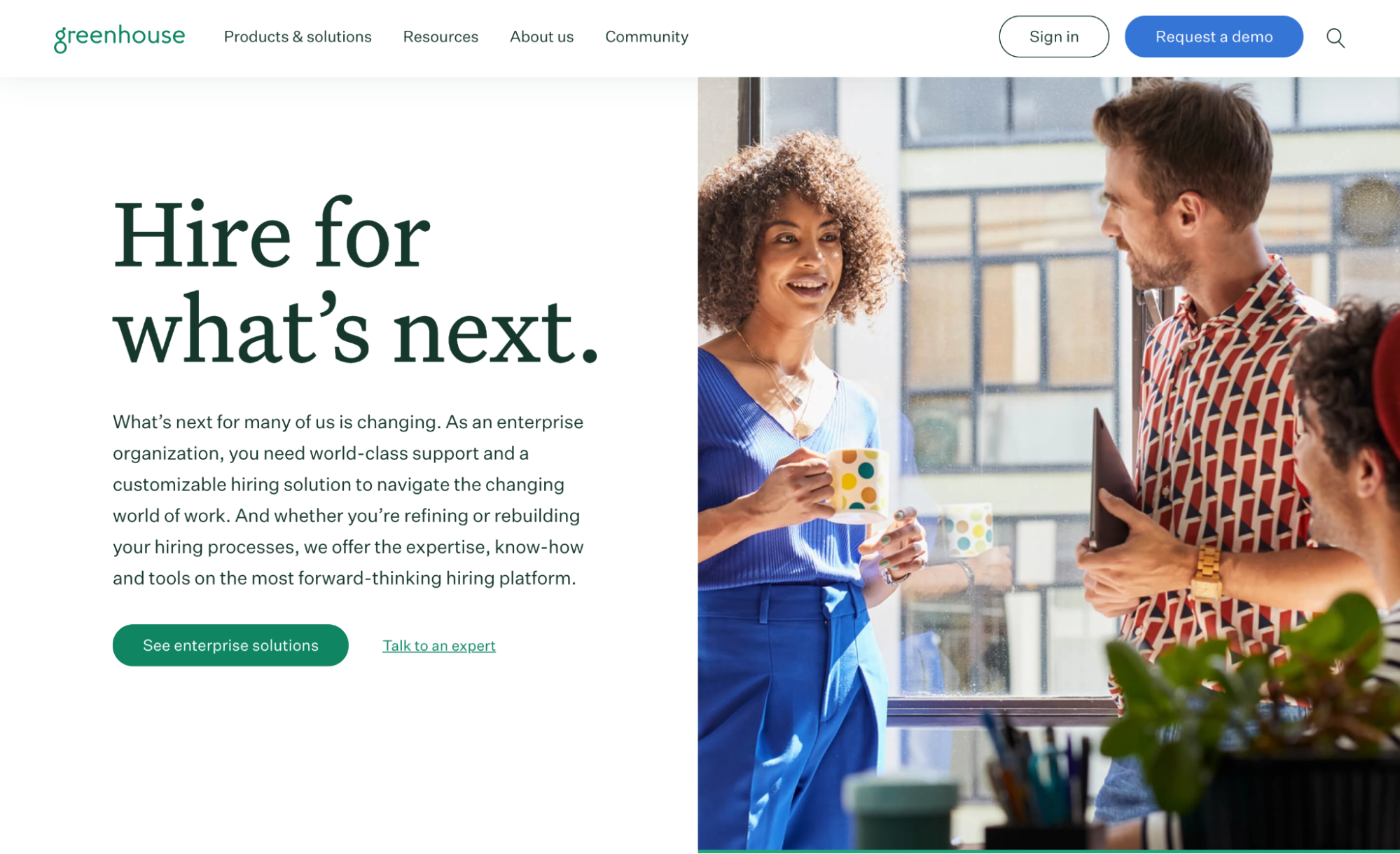Here is the cleaned-up and detailed descriptive caption for the image from the Greenhouse website:

---

The screenshot from the Greenhouse website displays a minimalist and professional design. The upper navigation bar, set against a white background, prominently features the Greenhouse logo in green lowercase letters. To the right of the logo, the main navigation options are listed in black text: “Products and Solutions,” “Resources,” “About Us,” and “Community.” Further to the right are two buttons: a white "Sign In" button with black text and a blue "Request a Demo" button with white text. A magnifying glass icon indicating the search function is also present.

The main body of the page is divided into two halves. The left half features a white background with impactful black text. At the top, in very large font, the headline reads, "Hire for what's next." Below this, in a smaller font, the text continues: "What's next for many of us is changing. As an enterprise organization, you need world-class support and a customizable hiring solution to navigate the changing world of work. And whether you're refining or rebuilding your hiring processes, we offer the expertise, know-how, and tools of the most forward-thinking hiring platform." Beneath this text, there is a green button with white text that reads "See Enterprise Solutions." To the right of this button is an underlined green link that says "Talk to an Expert."

The right half of the main section reveals an image showcasing three individuals in what appears to be an office setting with a large sunlit window and a building visible in the background. From left to right, the individuals are: 
1. A smiling Black female with reddish-brown curly hair, wearing a gold necklace, a short-sleeved blue V-neck top, and blue trousers. She is holding a coffee mug adorned with orange, blue, and yellow spots in her right hand and has a bracelet or watch on her left wrist.
2. To her right is a Caucasian male with short brown hair and a light beard, looking at her in profile. He is wearing a collared T-shirt with a blue triangle and red stripes pattern, a gold watch on his left wrist, and appears to be holding a triangular object.
3. The third individual is another male, visible from the side, with curly brunette hair, smiling and wearing a red hat and a black striped white shirt. 

In the blurred foreground, there is a green succulent plant container holding pens or brushes alongside another green round container with a light blue top.